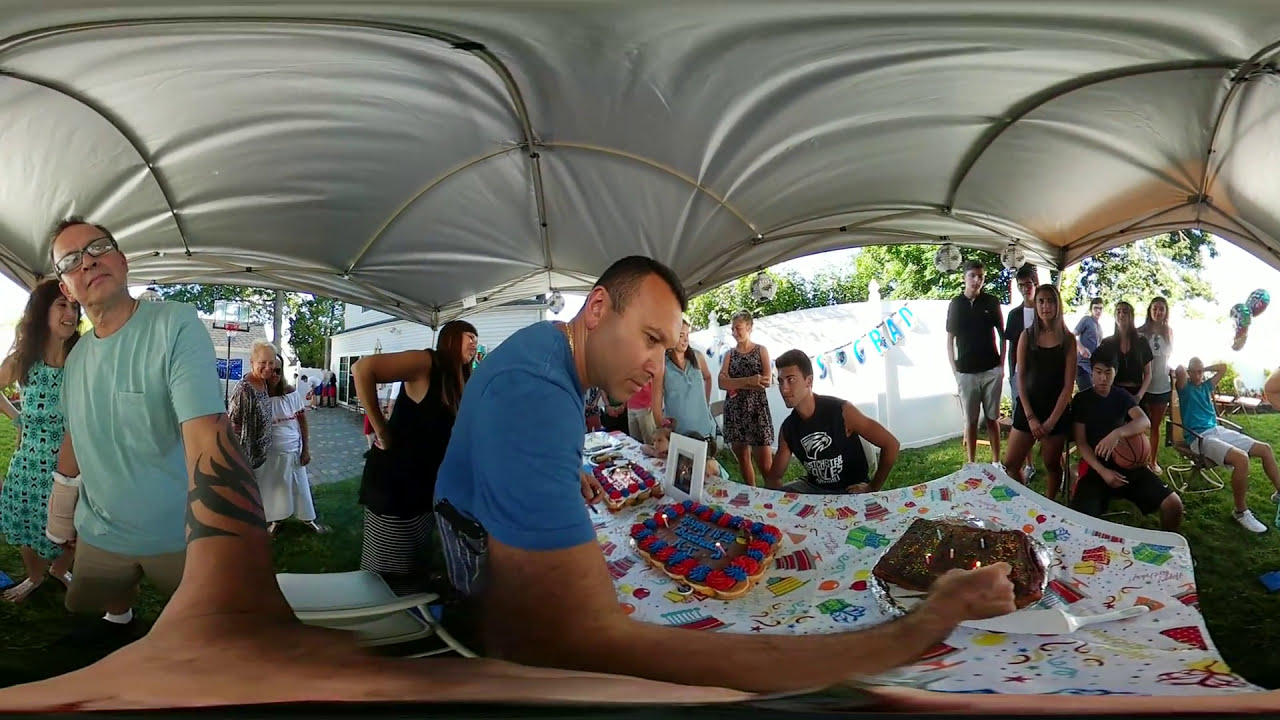This photograph captures a vibrant outdoor celebration set in a spacious suburban backyard during a bright, sunny day. Central to the scene is a large table adorned with a fun, colorful tablecloth featuring green, red, yellow, and other bright designs; it holds three cakes, two of which have candles. A man in a blue t-shirt with glasses, who seems to have a cast on his right arm, is seen lighting candles on a chocolate cake, flanked by another cake with red and blue icing and a third adjacent cake. A man with a tribal tattoo and pale blueish-green shirt stands to the left, smiling, and a woman in a similar blueish-green dress smiles behind him. 

The festivities are shaded under a large white tent or pavilion crowded with a diverse group of Caucasian individuals, ranging from children to the elderly. To the right, a boy holding a basketball can be seen, and an elderly lady is situated in the far left-hand corner. The scene is set against a backdrop of green grass, a white fence, a basketball hoop, and leafy green trees, confirming the summer season. The sky is partially visible, suggesting a middle-of-the-day lighting. The image appears slightly distorted, hinting at a 360-degree panoramic view, capturing the essence of a joyful gathering, potentially a birthday or a graduation party.